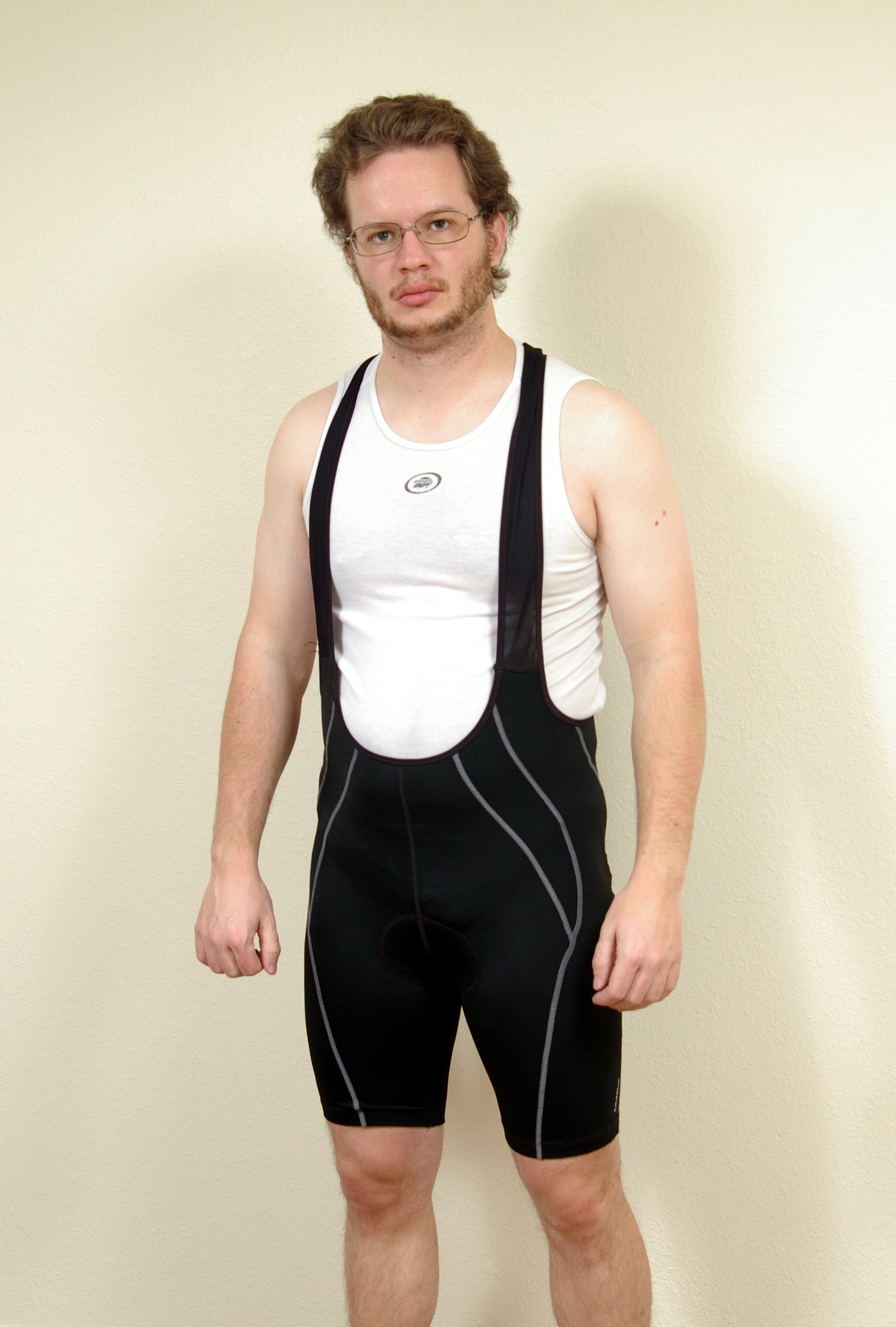A man is pictured wearing a one-piece wrestling or bodybuilding outfit. The ensemble features black suspenders and tight, knee-length shorts made from a stretchy material. Underneath, he sports a sleeveless white t-shirt (often referred to as a "Dago Tee") with a scoop neck and a small black round emblem on the upper chest. The shorts are adorned with light gray stripes running down the front and sides. His arms are bare and relaxed at his sides, revealing light hair on his legs and a pale complexion with a faint farmer's tan, along with a few freckles on his left upper arm.

The man has medium brown wavy hair, a short mustache, and a bit of a beard with some whiskers on his neck, adding to his casual appearance. He wears square wire-framed glasses, which could be for reading or distance. His expression is neutral, and he gazes forward as if posing for the photograph, with natural-colored lips and an overall calm demeanor.